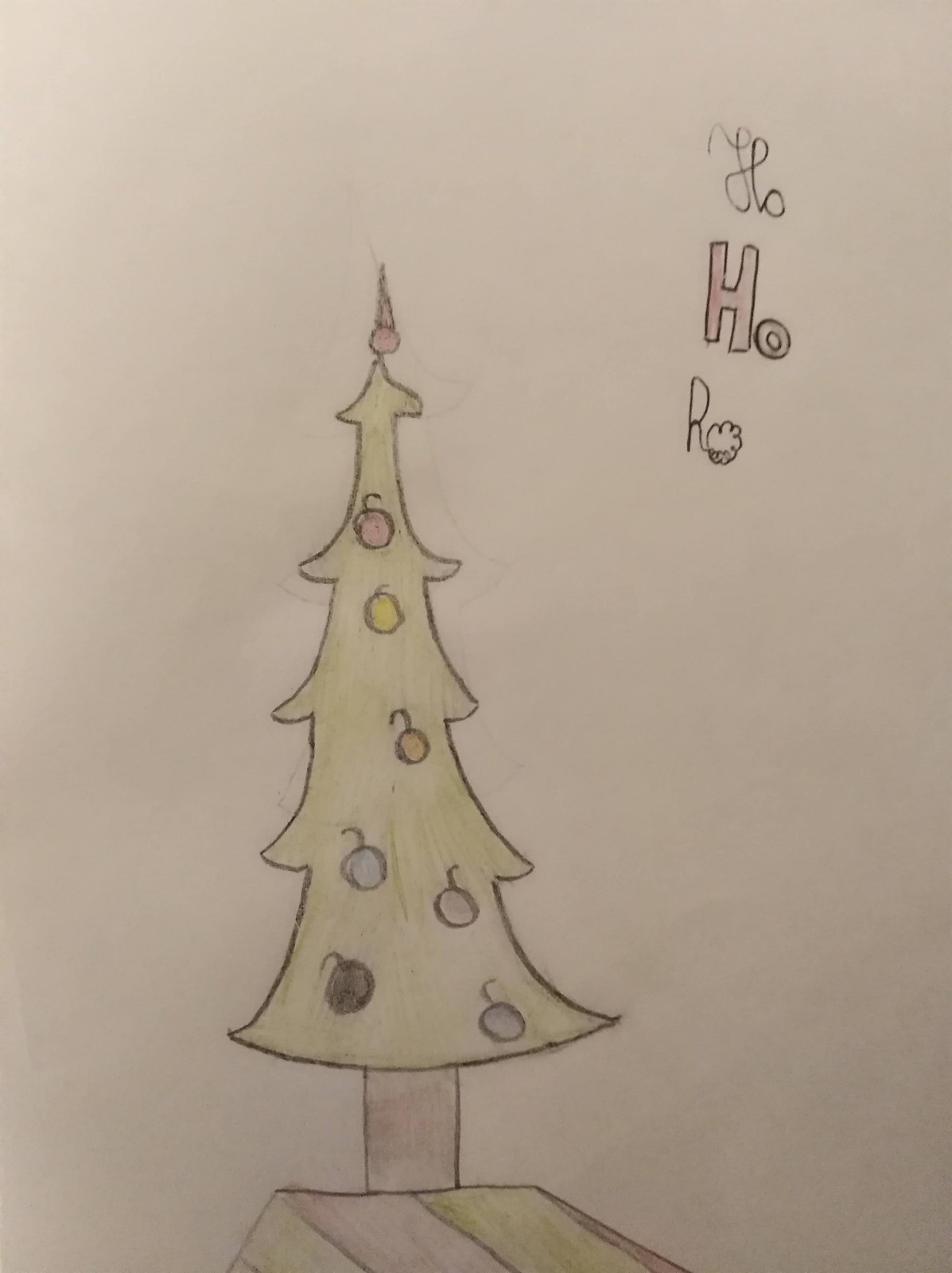This image is a child's drawing of a Christmas tree, rendered on a white sheet of paper. The Christmas tree itself is narrow and outlined in a black pencil, filled in with a green colored pencil. The tree is adorned with circular ornaments in different colors; noticeable ones include red, yellow, blue, black, and brown. These ornaments have visible hooks, suggesting a realistic touch. At the top of the tree is a peculiar ornament—round with a point protruding from it, unlike a traditional star or angel.

The tree stands on a base which could be mistaken for either a two-tone present or a peaked roof, faintly colored in brown and green/yellow tones. The trunk of the tree is brown, colored neatly with a colored pencil. 

In the top right corner of the drawing, there's a festive inscription reading "Ho Ho Ro" or potentially "Ho Ho Rho," with each "Ho" positioned on separate lines and outlined in different colors, possibly red. The last "Ho" is abbreviated or altered, morphing into what looks like a decorative element resembling a flower or a cloud. The entire scene maintains a simple, whimsical charm typical of a child's artwork, capturing the spirit of Christmas in a colorful and imaginative way.